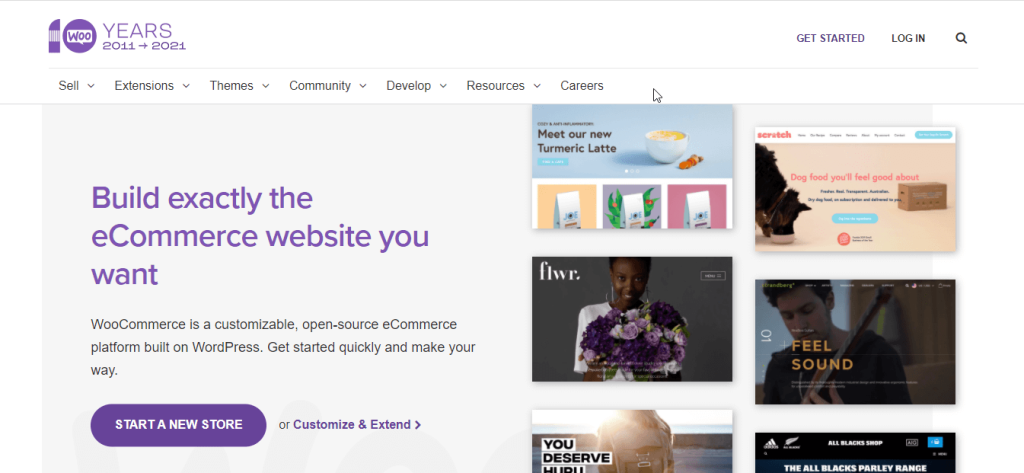**Screenshot from WooCommerce E-Commerce Platform Website**

The screenshot captures the homepage of the WooCommerce website, a platform allowing users to construct custom e-commerce websites through a simple, intuitive, point-and-click interface. The site has a clean and aesthetically pleasing design, primarily utilizing shades of purple.

**Header Section:**
- The top left corner features the WooCommerce logo in purple, celebrating their 10th anniversary with the text "Woo, 10 years 2011 - 2021."
- The top right corner includes a "Get Started" button, a "Login" button, and a search box.

**Navigation Menu:**
- Below the header, there is a horizontal navigation menu with the following options: Sell, Extensions, Themes, Community, Develop, Resources, and Careers.

**Main Content Section:**
- The left side of the main content area contains informative text about the platform. In a stylish purple font, it states, "Build exactly the e-commerce website you want." Beneath this headline, there is a smaller description that reads, "WooCommerce is a customizable, open-source e-commerce platform built on WordPress. Get started quickly and make your way."
- Directly below the description text, there is a purple button with white text labeled "Start a New Store or Customise and Extend," offering users options to either create a new store or modify an existing one.

**Visual Examples:**
- The right side of the page displays six images, which are screenshots of various e-commerce stores created using the WooCommerce platform, showcasing the diverse and customizable designs possible with the tool.

Overall, the screenshot provides an inviting and informative overview of the WooCommerce website, emphasizing the platform's ease of use and customization capabilities.